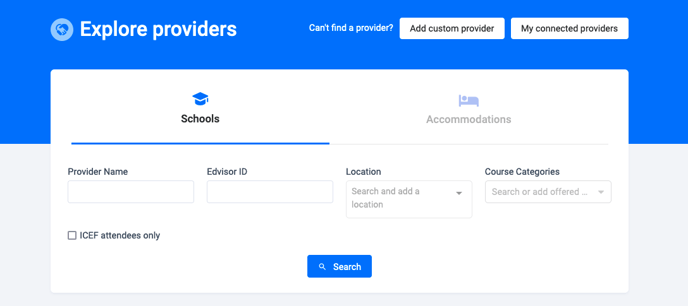Screenshot of a website interface with a predominantly blue and white color scheme. The background is primarily white with blue details, including a blue banner at the top. The banner features a logo of two hands shaking, followed by the text "Explore Providers" in white. Below the banner, there are two white buttons labeled "Add Custom Provider" and "My Connected Providers."

The webpage includes two menu options: "Schools" and "Accommodations," with "Schools" currently selected and highlighted by a blue underline. Underneath the menu options, there are free text boxes for "Provider Name" and "EdeVisorID." Adjacent to these text boxes, there are drop-down menus for "Location" and "Course Categories." The "Location" drop-down menu prompts users to "Search and add a location," while the "Course Categories" drop-down menu contains the partially visible placeholder text "Search or add offered..."

On the left-hand side below the drop-down menus, there is an unchecked tick box labeled "ICEF attendees only." The interface is completed with a centrally aligned blue search button at the bottom.